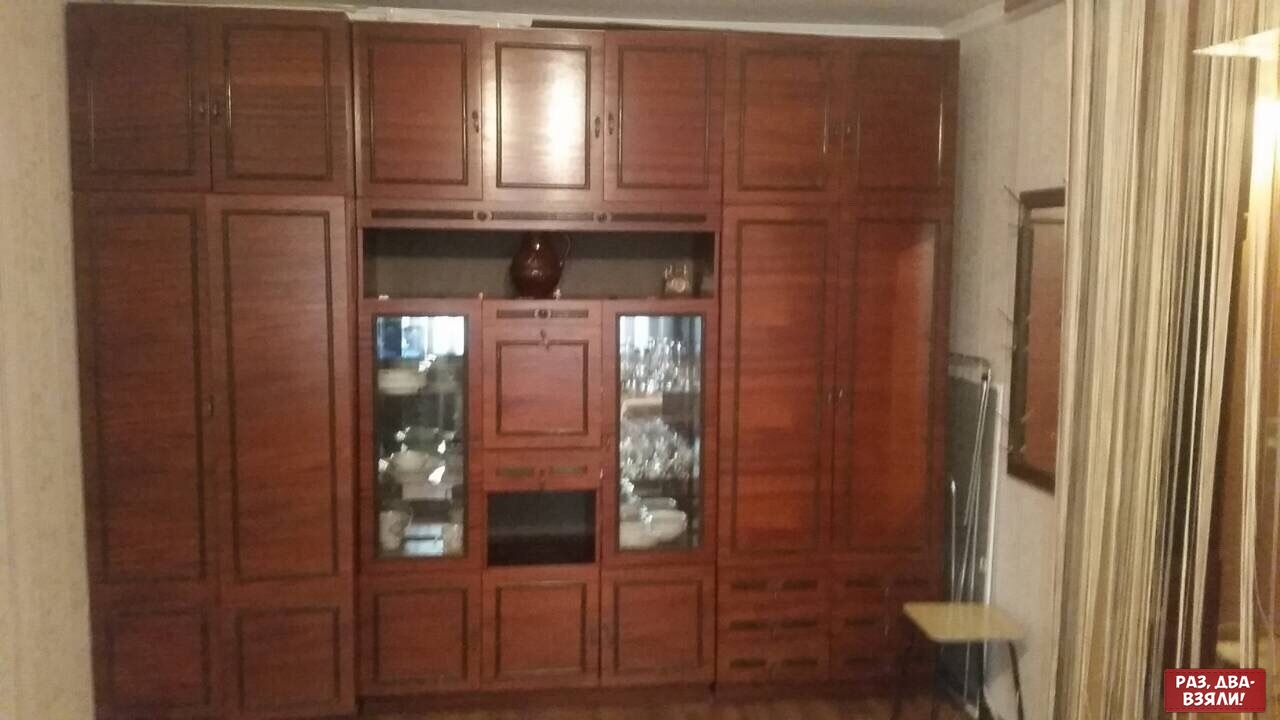This photograph captures the inside of a modest bedroom, possibly a hotel room, with a drab ambiance dominated by creamy tones. The wallpaper seamlessly matches the curtains, reinforcing the neutral, somewhat uninspired decor. The focal point of the room is an extensive and rather unattractive piece of furniture that spans the entire back wall from floor to ceiling. This colossal brown laminate wardrobe is divided into three main sections.

On the left side, it features a full-height wardrobe with two large doors, topped by two cupboards and accompanied by smaller storage spaces below. The central section is more intricate, hosting multiple smaller cupboards and glass shelving designed for display purposes. These shelves showcase an assortment of glasses and a few pieces of crockery. The right side mirrors the left, but instead of smaller storage boxes at the bottom, it is fitted with several drawers. The upper part of the wardrobe includes eight cabinets—two on each end and four in the middle. An open space in the middle section displays a vase and a glass, adding a slight decorative touch amidst the overwhelming functionality of this massive cabinet structure.